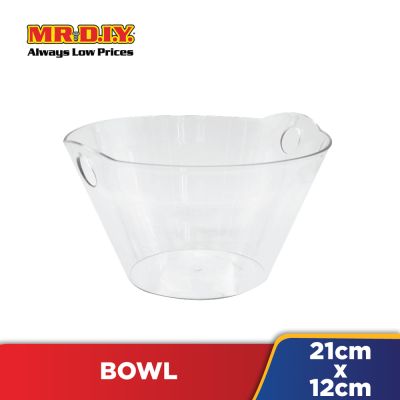The image is a professional advertisement for a transparent bowl, featuring prominent branding and detailed product specifications. The bowl, with an inverted cone shape where the base is narrower than the top opening, is centrally positioned against a plain white background. Notably, there are two small holes near the rim on the side of the bowl. Situated in the upper left corner is the "Mr. DIY" logo, written in bold red letters with yellow and black outlines, and accompanied by the tagline "Always Low Prices" in black text. A small silver screw graphic is embedded between "Mr." and "DIY." Below the bowl, a horizontal red rectangle banner features the word "BOWL" in white capital letters. To the right of this banner, a blue rectangle with a yellow stripe bears the bowl's dimensions, "21cm x 12cm," written in white text. The precise placement and detailed design elements suggest this image is aimed at advertising the bowl as an affordable product available at Mr. DIY stores.